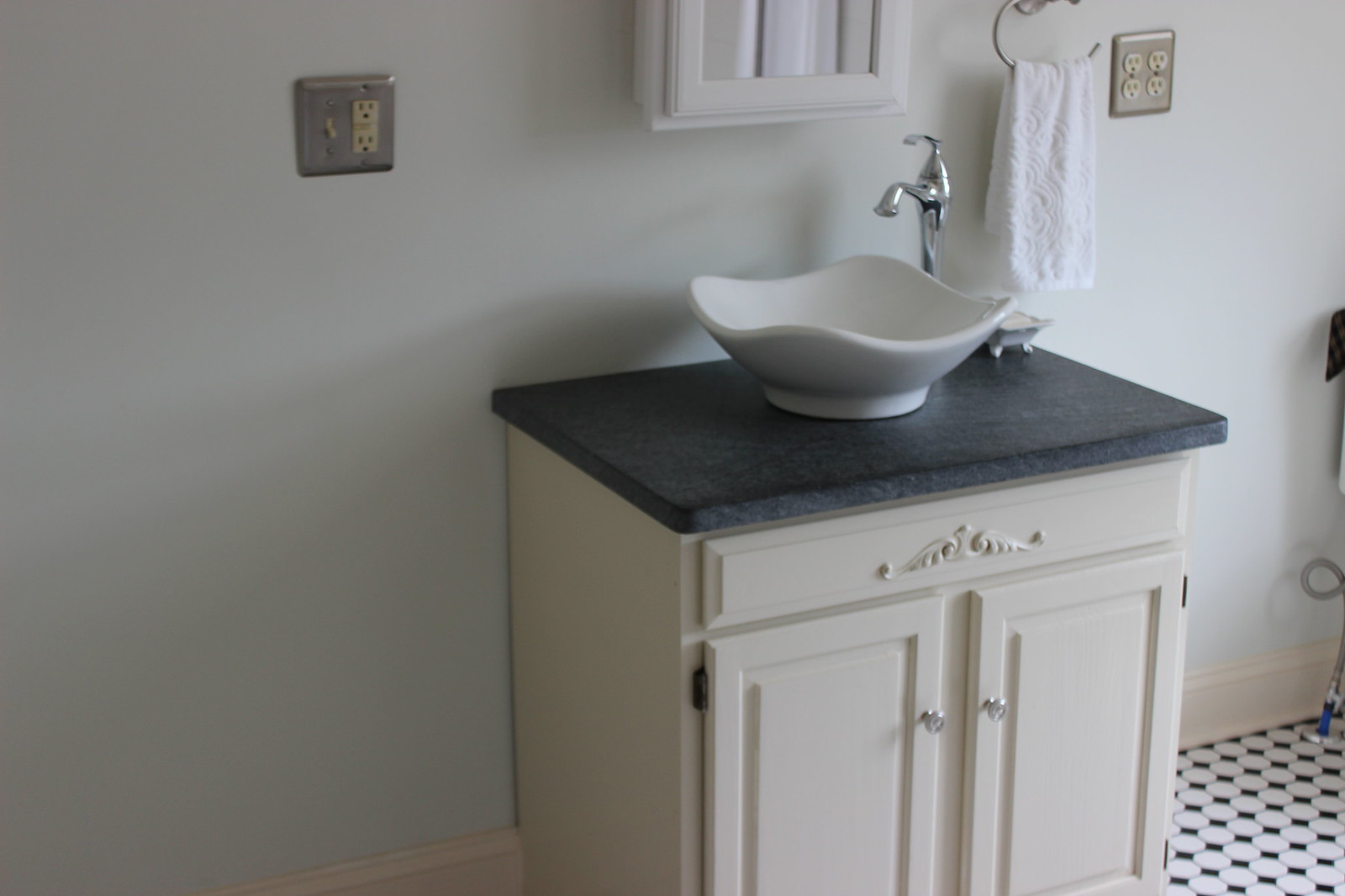The photograph captures a meticulously arranged bathroom interior with a minimalist and modern aesthetic. The dominant white wall serves as a pristine backdrop, against which various elements of the room stand out vividly. From the right side of the frame, a light source casts soft shadows to the left, highlighting the details of the setting.

Prominently featured on the white wall are two silver plates covering electrical fixtures. On the left side, one plate conceals two electrical sockets and a single light switch, which is positioned downward. On the right side, a larger silver plate encases four electrical sockets arranged in a square pattern—two at the top and two at the bottom.

Central to the composition, partially cut off at the top, is a white medicine cabinet protruding slightly from the wall, with a reflective mirror embedded in its door. Below the cabinet sits a sophisticated vanity, characterized by a dark countertop that prominently features a bowl-like sink. Adjacent to the sink is a sleek silver tap and a contemporary gray soap dish containing a bar of soap.

Mounted on the wall is a towel rack designed in a distinctive C-hook form, holding a neatly folded white towel. The vanity’s base is cream-colored, complementarily offset by the silver handles on its dual doors. The floor below is an intricate pattern of small black and white tiles, culminating at the wall with a cream-colored baseboard trim that adds a subtle contrast to the overall décor.